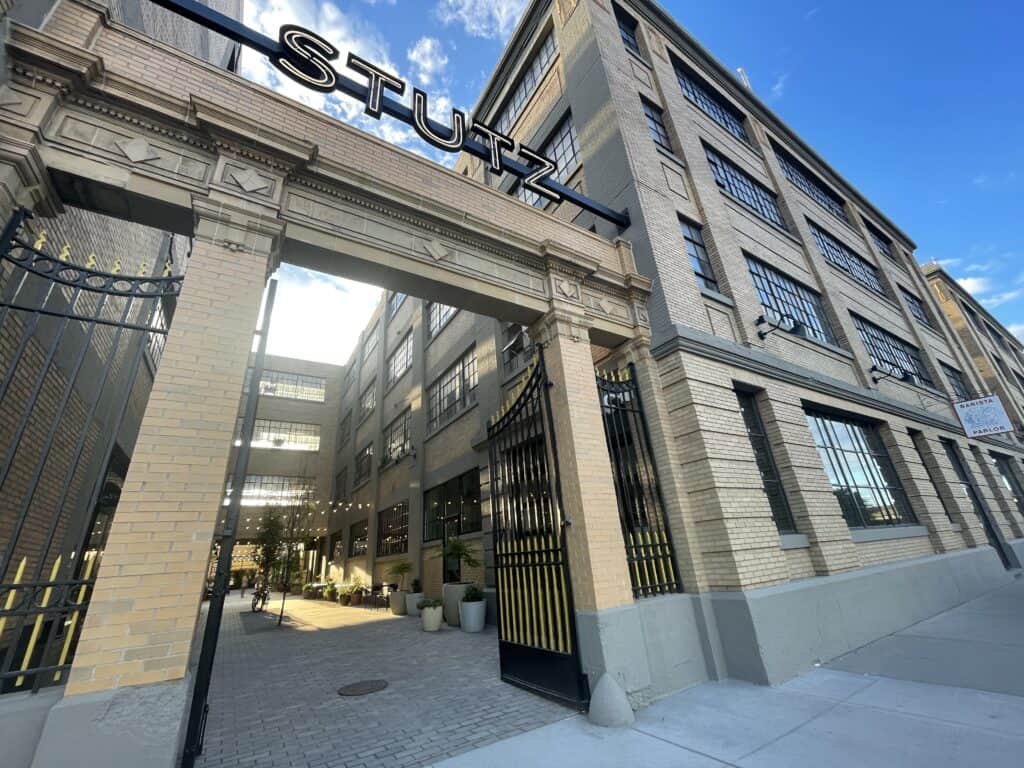This photograph captures the entrance to a courtyard situated between two towering brown brick buildings. The shot is taken from the bottom left perspective, looking upward towards the bright blue sky dotted with a few fluffy white clouds. The entrance features an archway marked by a sign that reads "Stutz," supported by large columns with intricate black and gold bars and a wrought iron gate that is open, invitingly swinging inwards. The arched entrance leads into a courtyard filled with sunlight and shade, adorned with numerous flower pots containing various plants. String lights crisscross above, adding a festive atmosphere to the space. The buildings, characterized by multiple black windows, have a connecting section elevated above the courtyard. Indistinct figures can be seen mingling in the background, adding life to the serene and picturesque scene.